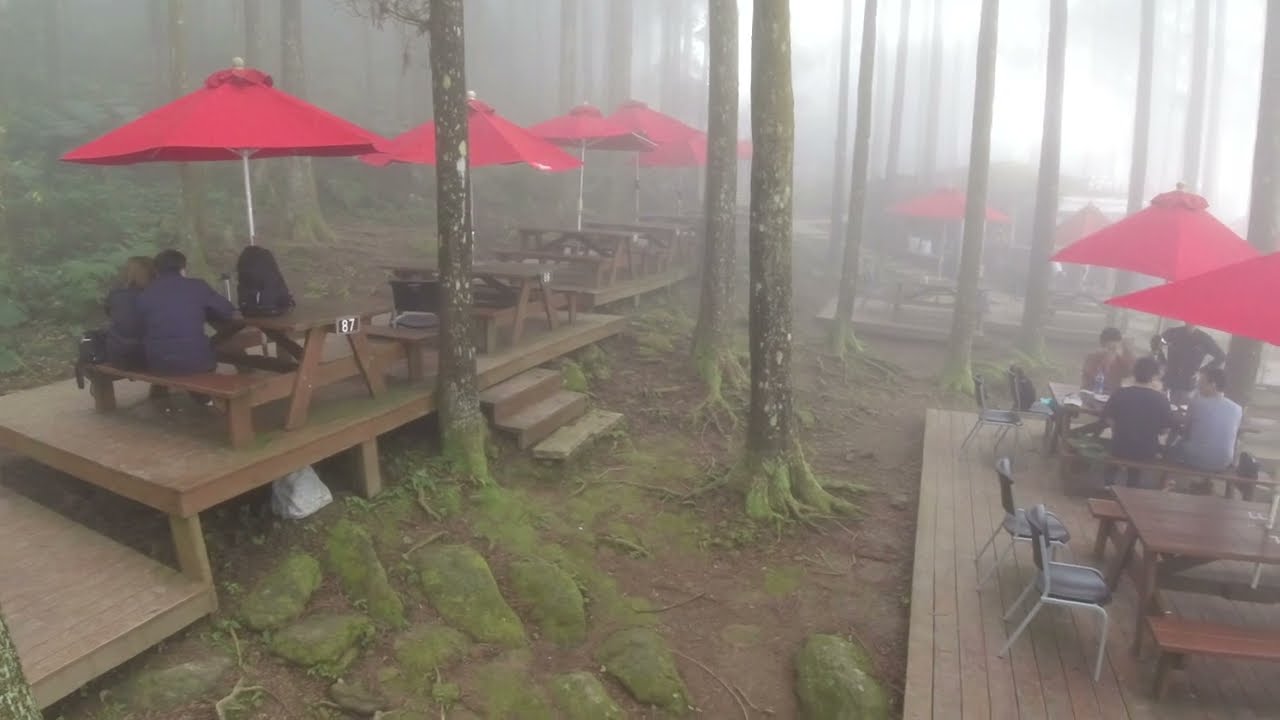This outdoor photograph captures a foggy, wooded area that seems to be a scenic, forested campground or a restaurant's outdoor seating section. Wooden decks are meticulously arranged around the trees, each supporting picnic bench tables topped with vibrant red sunshade parasols, distinguished by their white stems. Moss clings to rocks and tree trunks, emphasizing the lush, green environment. Situated among this dense greenery and scattered brown earth, several groups of diners are visible, some enjoying meals while others appear to be resting. Most of the tables remain empty, accentuating the stillness of the fog that blankets the background. The dense haze limits visibility, adding a mystical quality to the scene, while bushes and leaves add to the naturalistic setting.